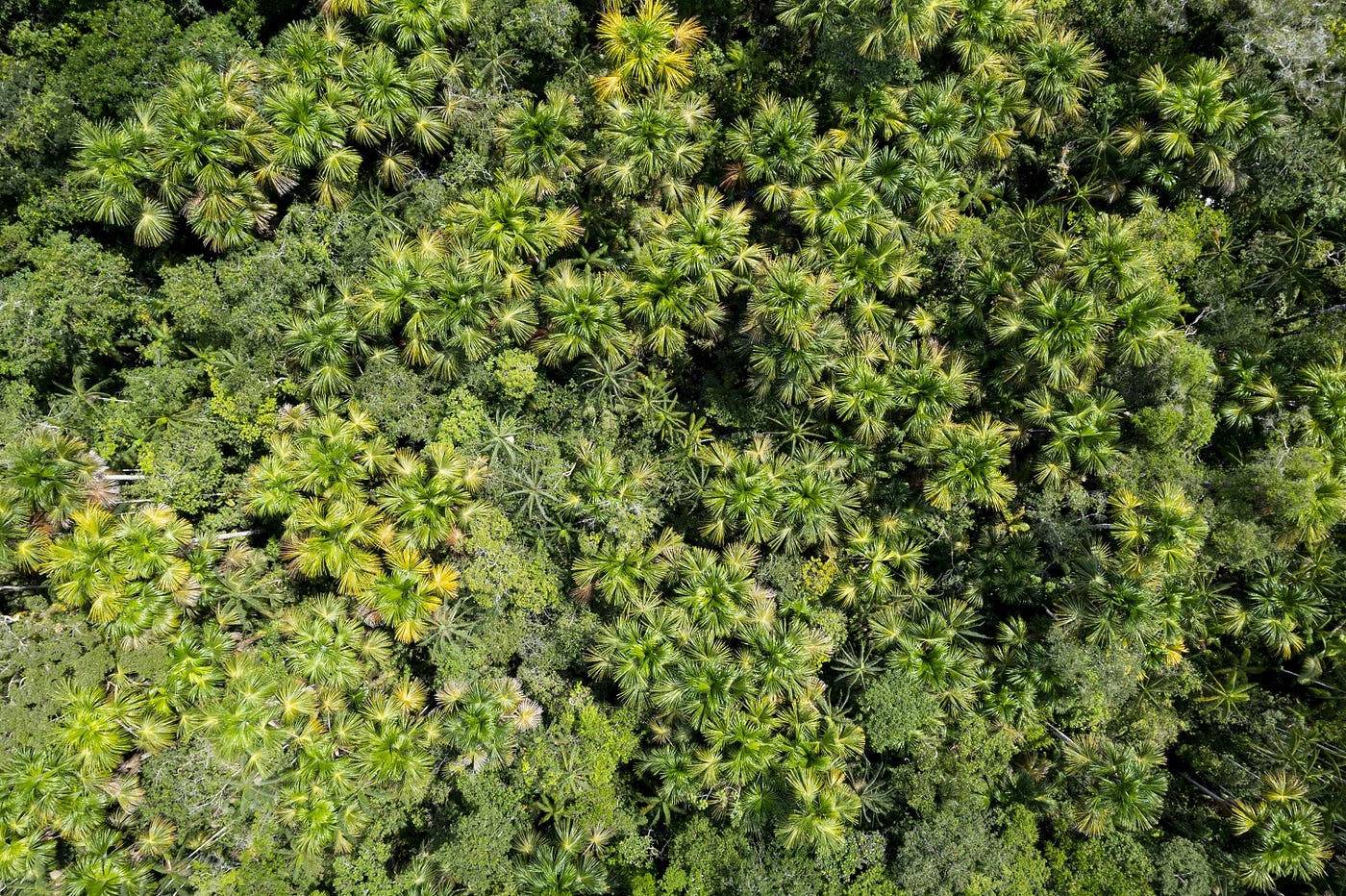This aerial photograph captures a lush, densely packed forest, possibly a rainforest, dominated by a vibrant, green canopy. From this high vantage point, the ground is completely obscured by a variety of trees, with a significant number of them appearing to be palm trees. The palm trees are characterized by their spiky, fan-shaped leaves that stand out in contrast to the other types of foliage. The canopy exhibits a rich spectrum of green shades, with some leaves tinged with yellow. Occasional darker patches and shadowy areas suggest the presence of tree trunks, especially along the bottom left and right corners of the image. There is a small spot of white at the top right, adding a minor element of contrast. The overall effect is a mesmerizing sea of green, with the distinct, airy arrangement of palm leaves interspersed throughout the dense forest.